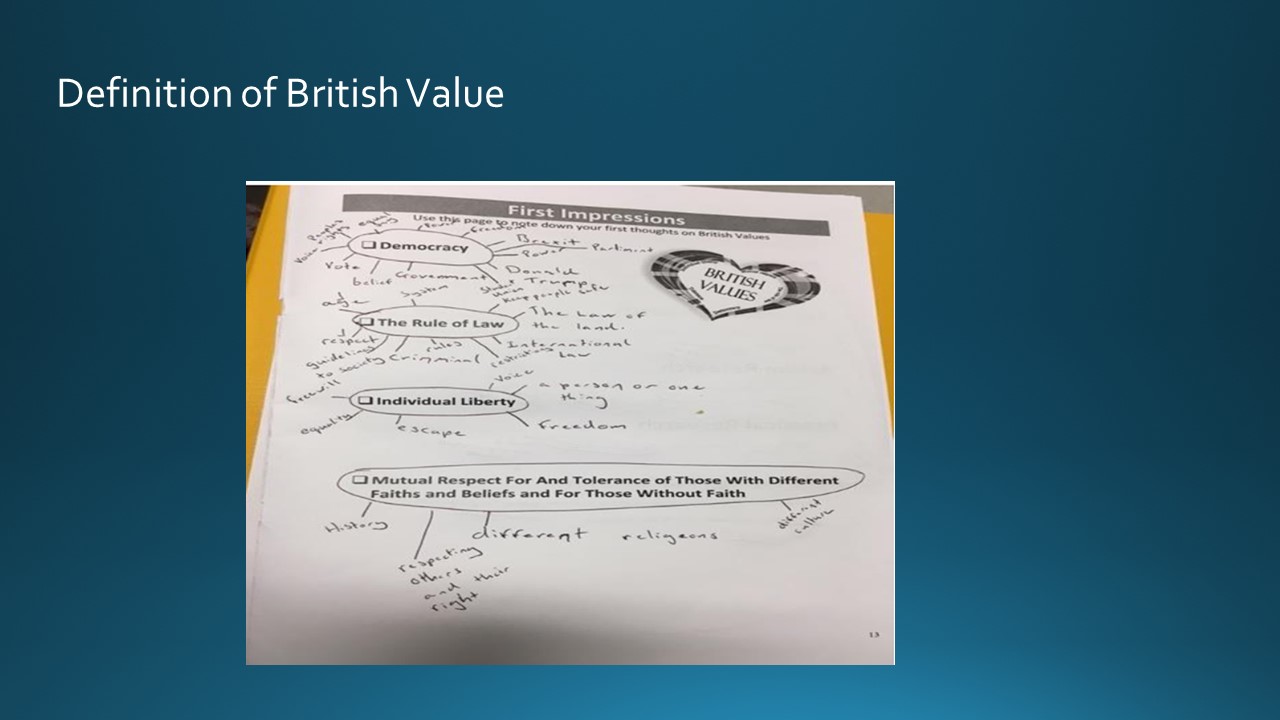The image showcases a white piece of paper set against a large, sky blue background. On the upper left corner of the blue background, white text reads "Definition of British Value." The paper itself, apparently torn from a yellow notepad, prominently features a black banner at the top with white text that states "First Impressions." Below this banner, the paper is organized into four sections, each labeled with a key British value: Democracy, the Rule of Law, Individual Liberty, and Mutual Respect for and Tolerance of Those with Different Faiths and Beliefs and for Those Without Faith. On the upper right corner of the paper, a black and white heart bears the text "British Values." These sections are intended for noting down initial thoughts on the respective values, and the student has written several pencil notes, though they are difficult to read. The entire layout suggests it's part of a school project focused on exploring and understanding British values.